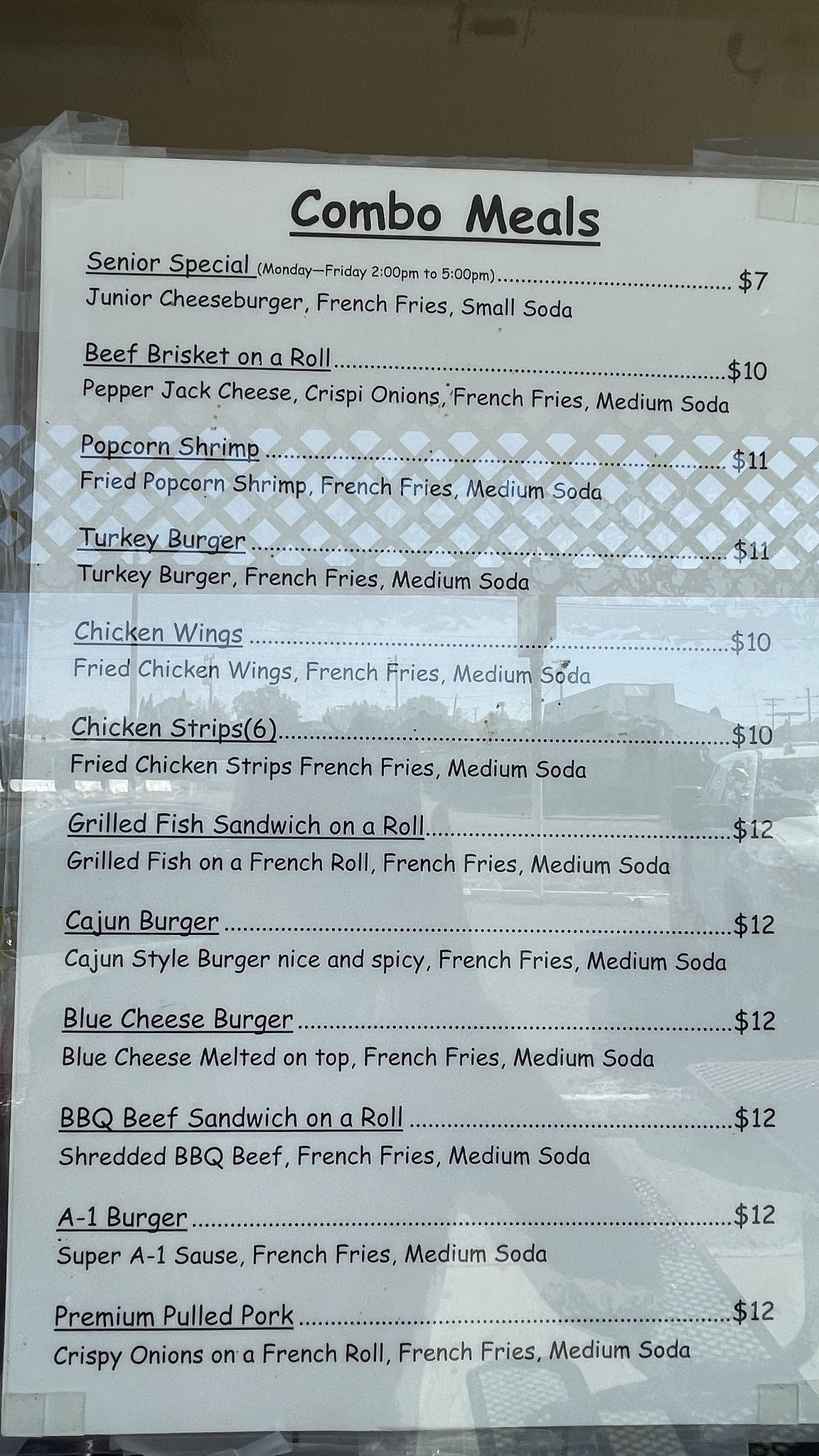A simple, monochrome menu is prominently displayed on a window, secured by layers of scotch tape at the top. The reflection on the window captures the image of a person and a metal picnic table with perforated seats and tabletop for drainage, situated just outside. Behind the table, a parked car and distant buildings are visible, adding context to the setting.

The menu itself is a white sheet encased in a plastic cover, detailing the available "Combo Meals." It advertises a "Senior Special" for $7, available Monday through Friday from 2 PM to 5 PM. The food items are listed in ascending order of price, starting with options like popcorn shrimp, turkey burger, chicken wings, and chicken strips. It also features grilled fish, a chicken sandwich on a roll, a Cajun burger, a blue cheese burger, a barbecued beef sandwich on a roll, and a "1" burger. The premium pulled pork, marked as the most expensive item, is priced at $12.